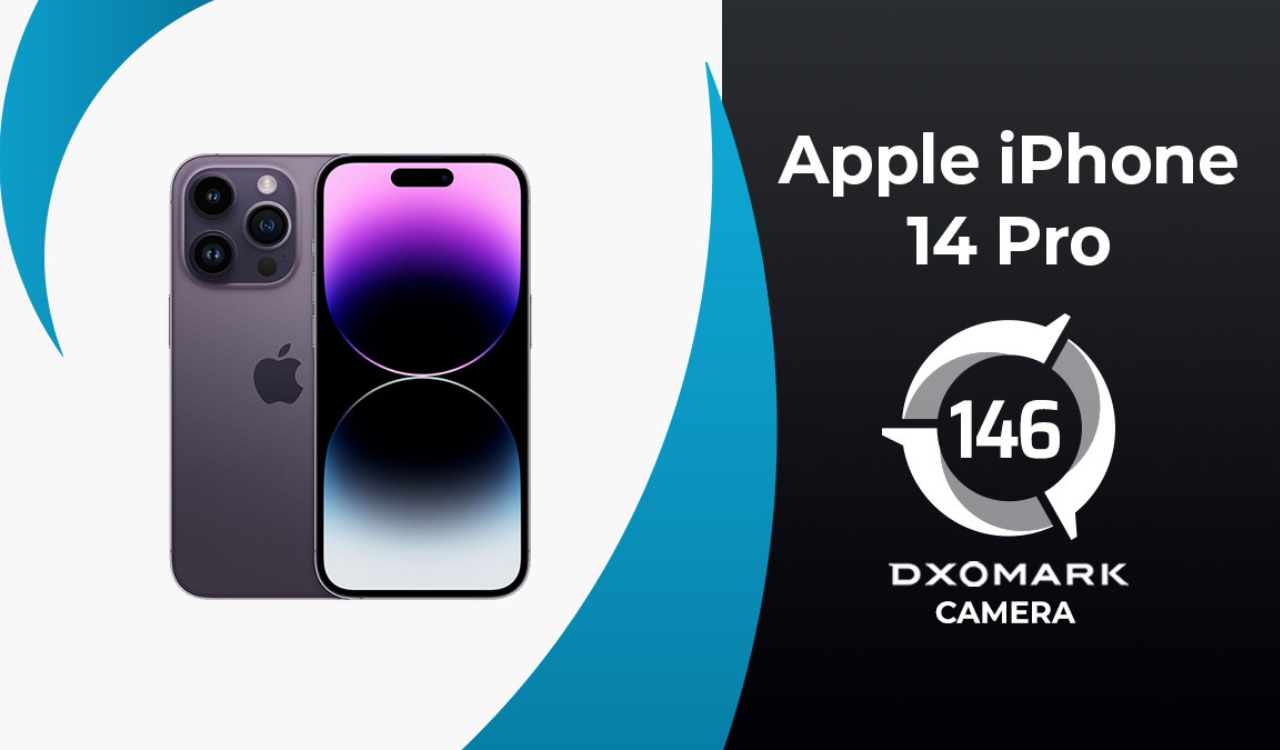This advertisement showcases the Apple iPhone 14 Pro from both its front and back perspectives. On the left side of the image, the phone is displayed to reveal its sleek design. The back of the iPhone 14 Pro is adorned with the Apple logo centered on its surface and features a sophisticated triple-camera system arranged within a square module. The color of the back is a stylish gray.

Meanwhile, the front screen of the phone boasts a stunning gradient that transitions from a pastel lavender at the top to a rich deep purple at the bottom. The center of the screen is adorned with an eye-catching artistic design consisting of two U-shaped patterns. The first U-shape starts with a black hue at the top and gently shifts to a baby blue, then a very light blue. The second U-shape mirrors this color progression and the bends of the two U’s are touching each other, forming an interesting visual harmony.

In the upper right corner of the image, there is a circular badge with slight extensions, prominently displaying the number "146" along with the text "DXOMARK Camera," indicating the impressive camera quality rating of the iPhone 14 Pro. This advertisement effectively highlights the elegant design and advanced camera capabilities of the Apple iPhone 14 Pro.